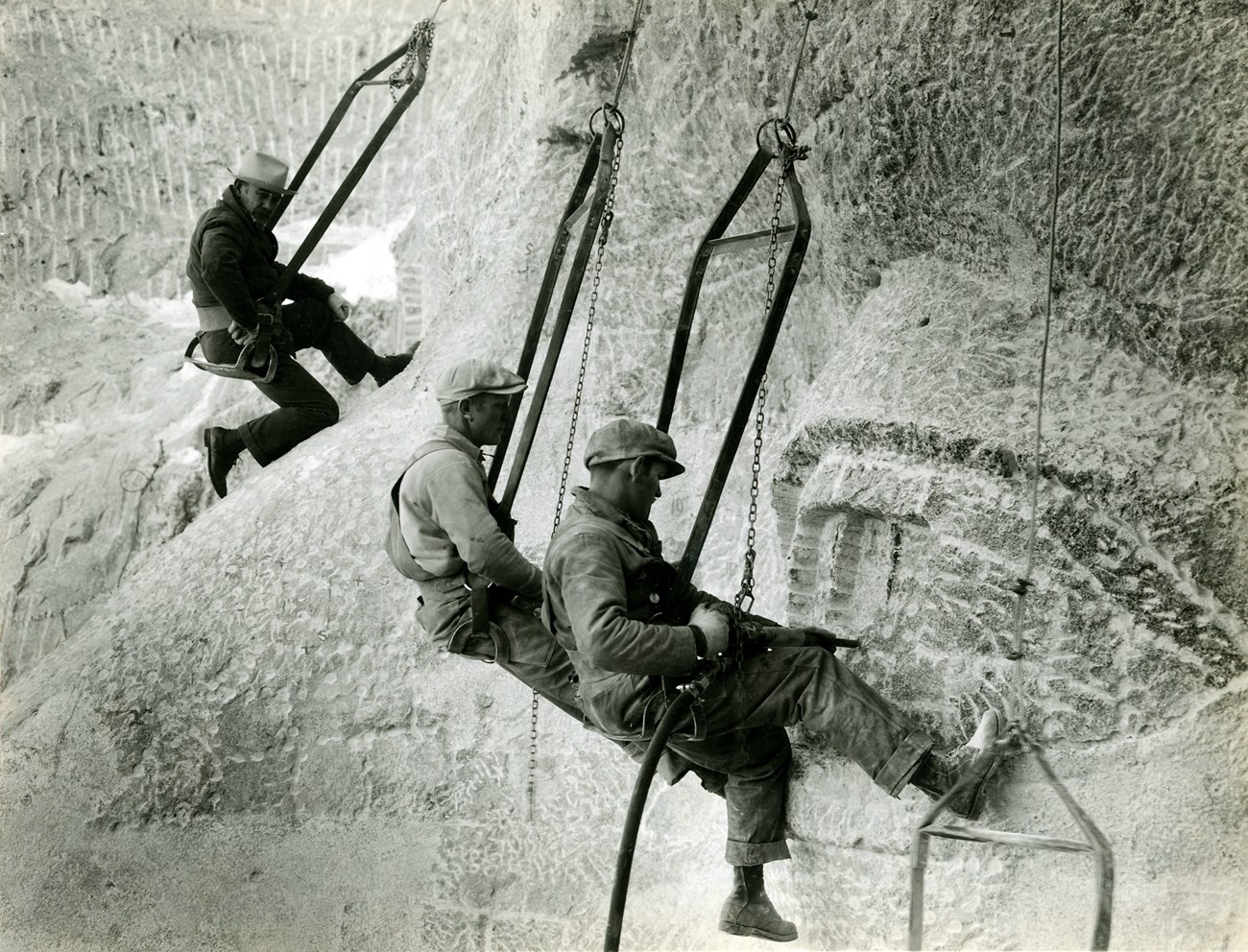In this black and white photograph, three men, appearing as professional workers or climbers, are suspended against a massive, textured rock formation. Dressed in military-style uniforms and safety gear, including hats, slacks, jackets, and boots, they are equipped with harnesses, metal chains, and wires. Each man is captured in profile, obscuring their faces, as they methodically scale the rock, suggesting a descent. Positioned towards the center of the landscape-oriented image, they are engaged in an activity that might involve tools or weapons. The rock's detailed surface adds depth to the scene, creating a dramatic and enigmatic atmosphere reminiscent of a historical or adventurous setting.